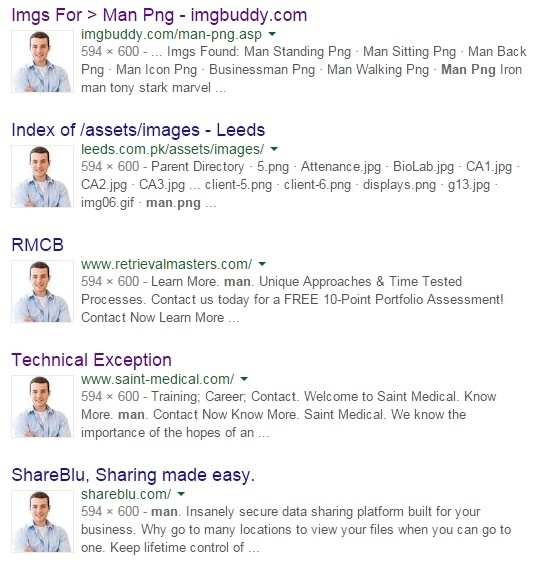In the image, the primary focus is a man standing confidently with his arms crossed over his chest. He is wearing a white t-shirt layered with a blue button-down shirt. His brown hair is neatly styled, and he is smiling warmly at the camera. The backdrop includes various text elements that distract from the main subject. At the top of the image, there is text that reads "images for man PNG" along with the website "imagebuddy.com". Below this, a list of search results is partially visible, including terms such as "man standing PNG", "man sitting PNG", "man back PNG", "businessman PNG", "man walking PNG", "man PNG", and even "iron man Tony Stark marble...".

Further down, there are additional references to image repositories and asset listings like "index of assets/images-leads" from leads.com, "RMCB" from retrievalmasters.com, "technical exception" from stmedical.com, and "ShareBlue sharing made easy" from shareblue.com. The repetition of these elements suggests the image might be a screenshot from an online image search or a website featuring multiple images of the same man in different postures. Despite the clutter of text, the man's cheerful demeanor and casual attire stand out as the primary focal point of the photograph.